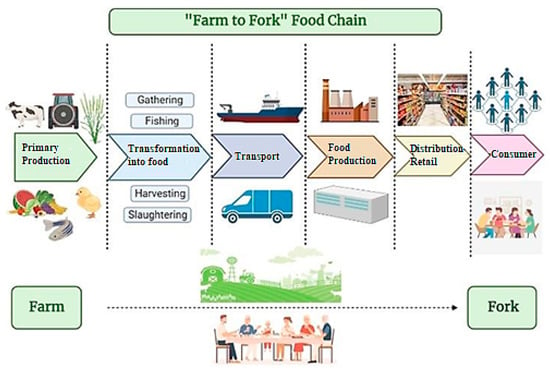This detailed infographic illustrates the "Farm to Fork Food Chain" with a clear, step-by-step visual representation on a white background. 

- **Title Bar:** The title "Farm to Fork Food Chain" is prominently displayed in dark green text on a light green highlighted bar.

- **Primary Production:** On the left, it begins with "Primary Production" signified by a green arrow and features drawings of a black and white Holstein cow, a green plant, and some fruits, fish, and a chick at the bottom.

- **Transformation into Food:** The next section, highlighted in blue, is labeled "Transformation into Food" and subdivides into four boxes, each labeled "Gathering," "Fishing," "Harvesting," and "Slaughtering."

- **Transport:** Following this, an arrow labeled "Transport" leads to images of a ship and a blue van illustrating the transportation phase.

- **Food Production:** Next is the "Food Production" stage, illustrated in brown, featuring a factory and a generic gray building.

- **Distribution Retail:** The process continues to “Distribution Retail,” with a supermarket illustration.

- **Consumer:** Finally, the chain ends at the "Consumer" stage, showing various people enjoying food.

Dotted lines separate each section, effectively outlining the sequence from primary production to the consumer's table, providing a comprehensive overview of how food travels from the farm to your fork.